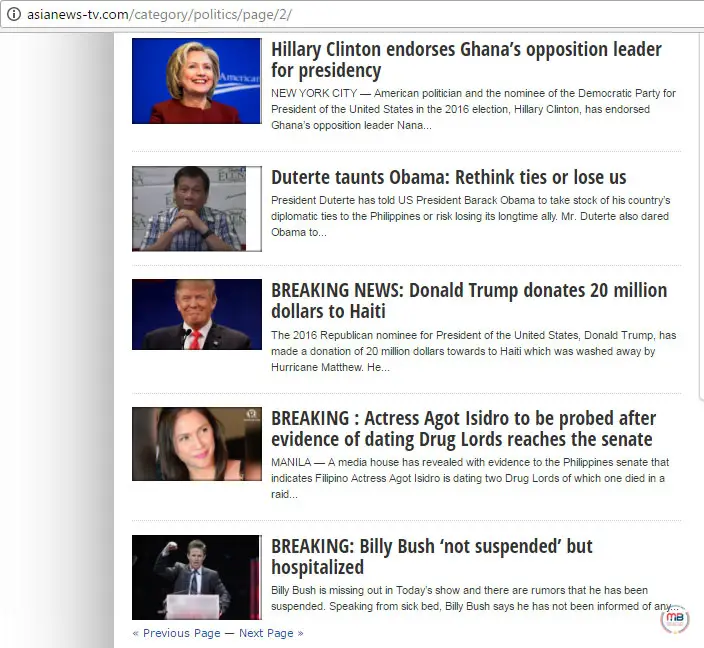This screenshot captures a section of political news articles, presumably from around 2016, based on the topics and individuals mentioned. The image is sourced from the website asianewstv.com, specifically from the Politics section on the second page. 

The articles are displayed in a vertical list, with five headlines presented in descending order:

1. **"Hillary Clinton Endorses Ghana's Opposition Leader for Presidency"** - Highlighting Clinton’s international political engagement.
2. **"Duterte Taunts Obama: Rethink Ties or Lose Us"** - Covering the strained ties between the Philippines and the US during Duterte's controversial leadership.
3. **"BREAKING NEWS: Donald Trump Donates $20 Million to Haiti"** - Announcing Trump's significant financial contribution to Haiti.
4. **"BREAKING: Actress Agathe Isidro to Be Probed After Evidence of Dating Drug Lords Breaches the Senate"** - Reporting an actress’s involvement in a scandal with criminal implications.
5. **"BREAKING: Billy Bush Not Suspended But Hospitalized"** - Providing an update on Billy Bush’s situation following a public controversy.

The context of the articles, featuring figures like Obama, Trump, and Clinton, situates the screenshot in the tumultuous political landscape of 2016.